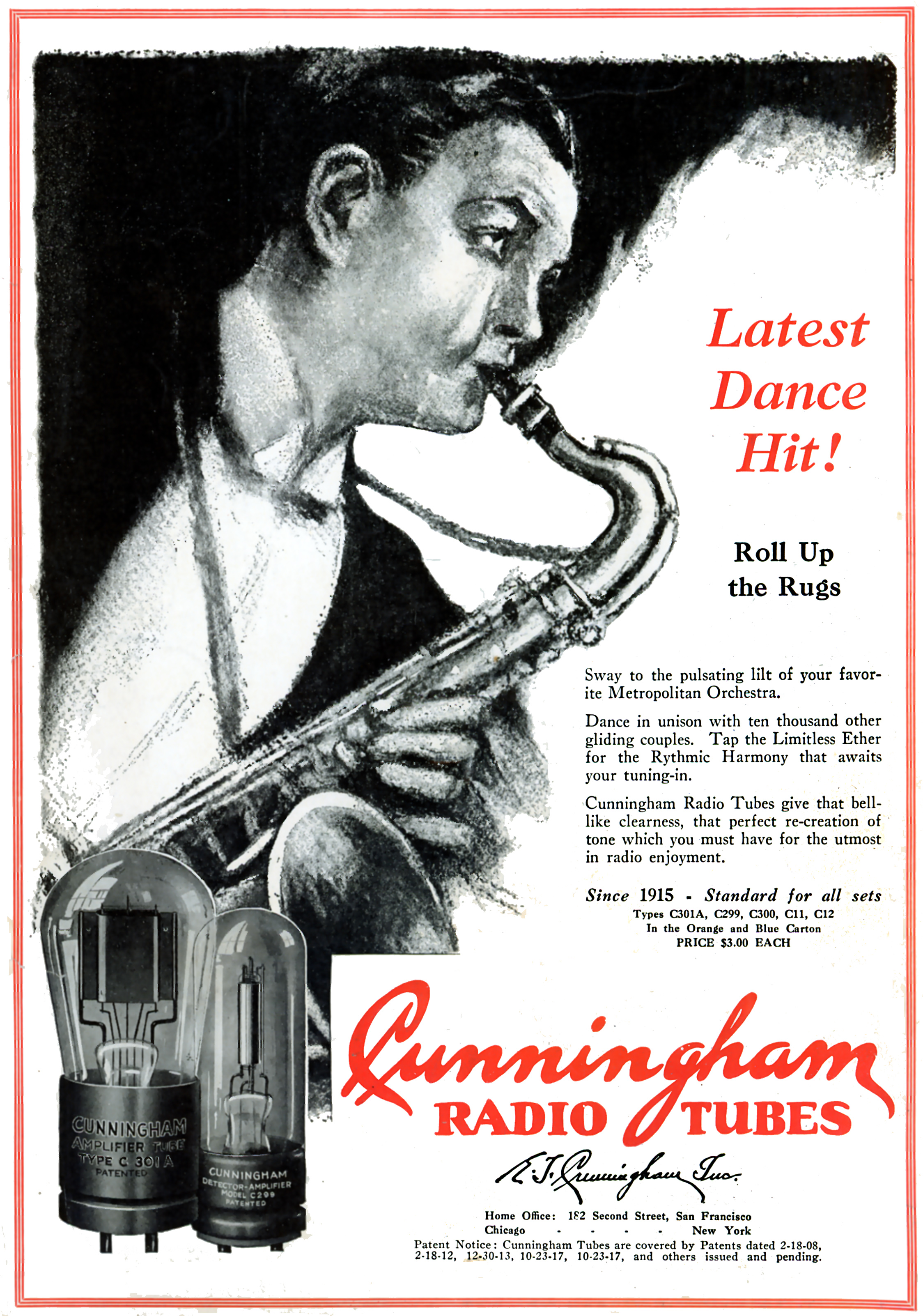This vertical, vintage magazine advertisement features a black-and-white illustration of a man in a tuxedo playing a saxophone, positioned at the top left of the image. This white man with a blurred black bowtie over a white shirt is blowing into the saxophone's black mouthpiece. The saxophone's body transitions from black to gray as it extends horizontally, curves upwards, bends down vertically, curls back upwards, and culminates in a large funnel shape adorned with numerous buttons along its vertical section, where the musician's hands rest.

Adjacent to the illustration is a series of promotional texts. In black, bold lettering, the ad announces, "Latest Dance Hit," followed by "Roll up the rugs" and, in smaller text, "Sway to the pulsating lilt of your favorite metropolitan orchestra. Dance in unison with 10,000 other gliding couples. Tap the limitless ether for the rhythmic harmony that awaits your tuning in." This is a nod to the social and communal experience of enjoying music over the radio. It continues to emphasize the product's superior quality by stating, "Cunningham radio tubes give that bell-like clearness, that perfect recreation of tone, which you must have for the utmost in radio enjoyment. Since 1915, standard for all sets.”

Below this descriptive text, the advertisement features the brand name "Cunningham" in red cursive, followed by "Radio Tubes" in red regular text. A signature, "RJ Cunningham," is also visible beneath these words. The visual composition is framed by a thin light-red stripe that outlines the entire rectangle.

In the bottom left corner of the advertisement, there are images of Cunningham radio tubes. The depicted cylinders have a black lower half and a clear upper half. The tube on the left is broader, with a slightly flared middle that arches into a dome at the top, while the tube on the right is narrower and rises straight up to a smaller dome.

This highly detailed ad not only emphasizes the latest dance hit and its associated joy but also highlights the high-quality radio tubes that promise an unparalleled auditory experience.